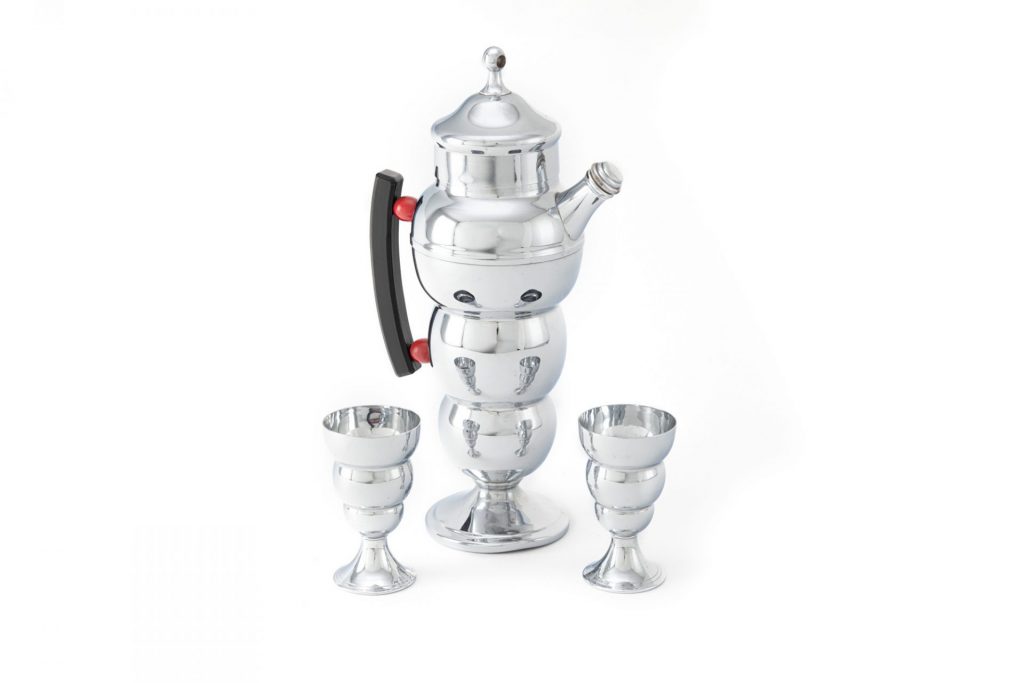The image features a sophisticated and futuristic tea set displayed against a plain white background. Central to the image is a reflective, silver metallic tea kettle resembling a reverse snowman, composed of three progressively larger, bulbous spheres stacked on top of each other. The kettle includes a black handle attached via distinctive red spheres, a small spout on the right side, and a lid with a round handle atop the widest sphere. Flanking the tea kettle on both sides are two elegantly designed metal cups, each with a form that narrows towards the bottom and opens wider at the top, similar in appearance to the kettle's spherical layers. The design combines function with a modern aesthetic, making it the focal point of the image. Subtle shadows from the cups add depth, completing the clean, minimalist composition.